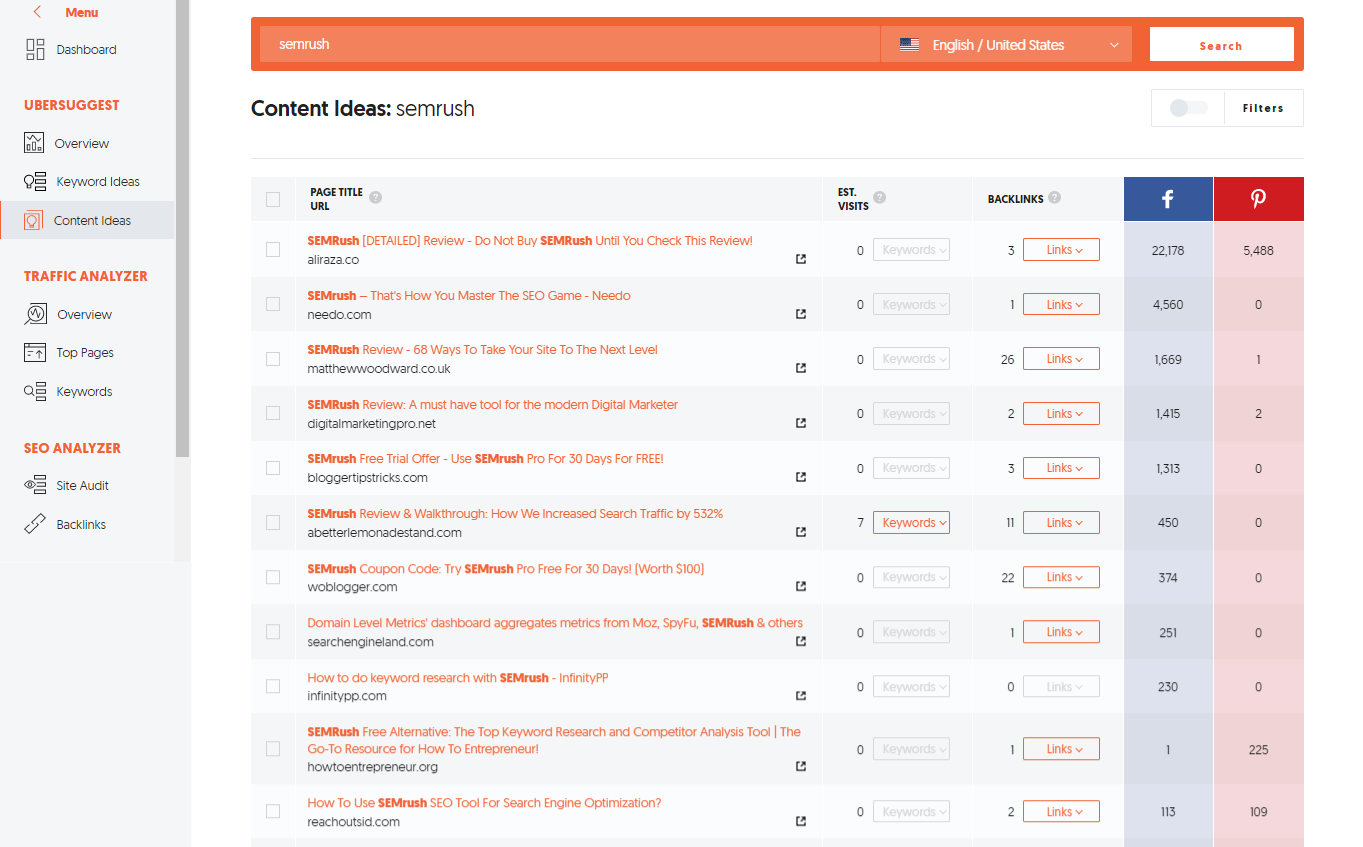A screenshot of a computer screen displaying SEMrush content ideas. The left side of the screen features a vertical navigation bar with a gray scrollbar, allowing users to browse through a multitude of information. The section titles are capitalized in orange, accompanied by small icons next to black text under each section. Dominating the right portion of the screen is a large, prominent orange header. To the far right edge of this header is a white search button. Below the header, the title "Content Ideas – SEMrush" is prominently displayed.

The main body of the screen consists of a sizable box displaying various titles written in bold orange text. Beneath each title is a snippet of black text, which appears to be web addresses. Adjacent to each title is a numeric value. Additionally, two columns, one blue with an "F" for Facebook and the other reddish with a "P" for Pinterest, list corresponding numeric statistics. Throughout the interface, there are rows with small selectable boxes, whose labels are unclear in this screenshot.